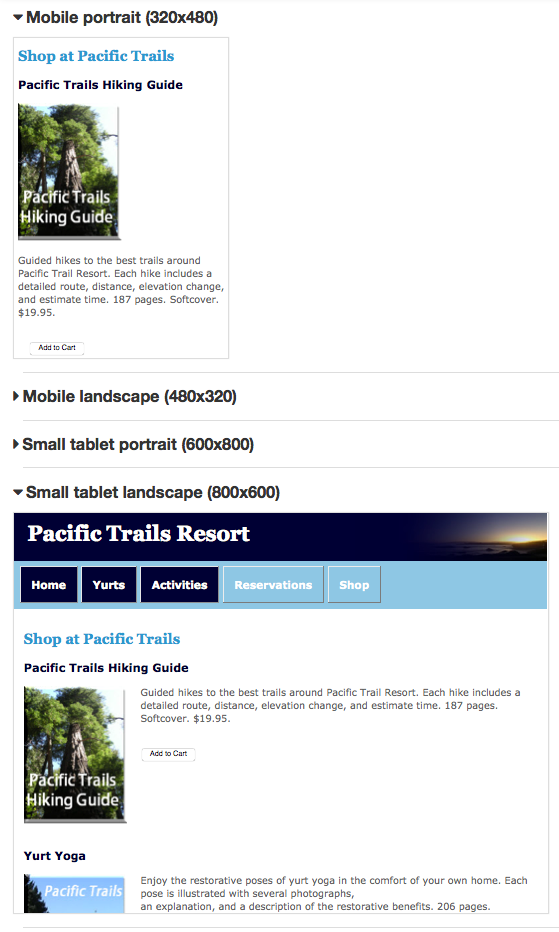This is a detailed descriptive caption for the provided image:

---
The image is a cropped screenshot of the download section for a hiking guide on the Pacific Trails website. The dimensions of the screenshot are 320x480 pixels, which is labeled "mobile portrait" in bold black letters at the top left corner. 

Directly below, there's a white box with "Shop at Pacific Trails" written in blue at the top left corner. Beneath this, in smaller black letters, it reads "Pacific Trails Hiking Guide." Adjacent, there's a square image displaying the text "Pacific Trails Hiking Guide" in white. Below this image, a short description of the hiking guide is provided alongside its price, $19.95. At the bottom left of this section, the text "Add to Cart" appears in very small black font.

Further below, the image indicates different device views including "mobile landscape," "small tablet portrait," and "small tablet landscape," with "mobile portrait" already expanded and "small tablet landscape" also expanded. 

For the "small tablet landscape" view, another square list is visible, starting with "Pacific Trails Resort" at the top left corner. At the bottom, various categories including "home," "yurts," "activities," "reservations," and "shop" are listed. Following this, "Shop at Pacific Trails" is repeated, showcasing thumbnails for both the Pacific Trails Hiking Guide and a Yurt Yoga Guide.
---